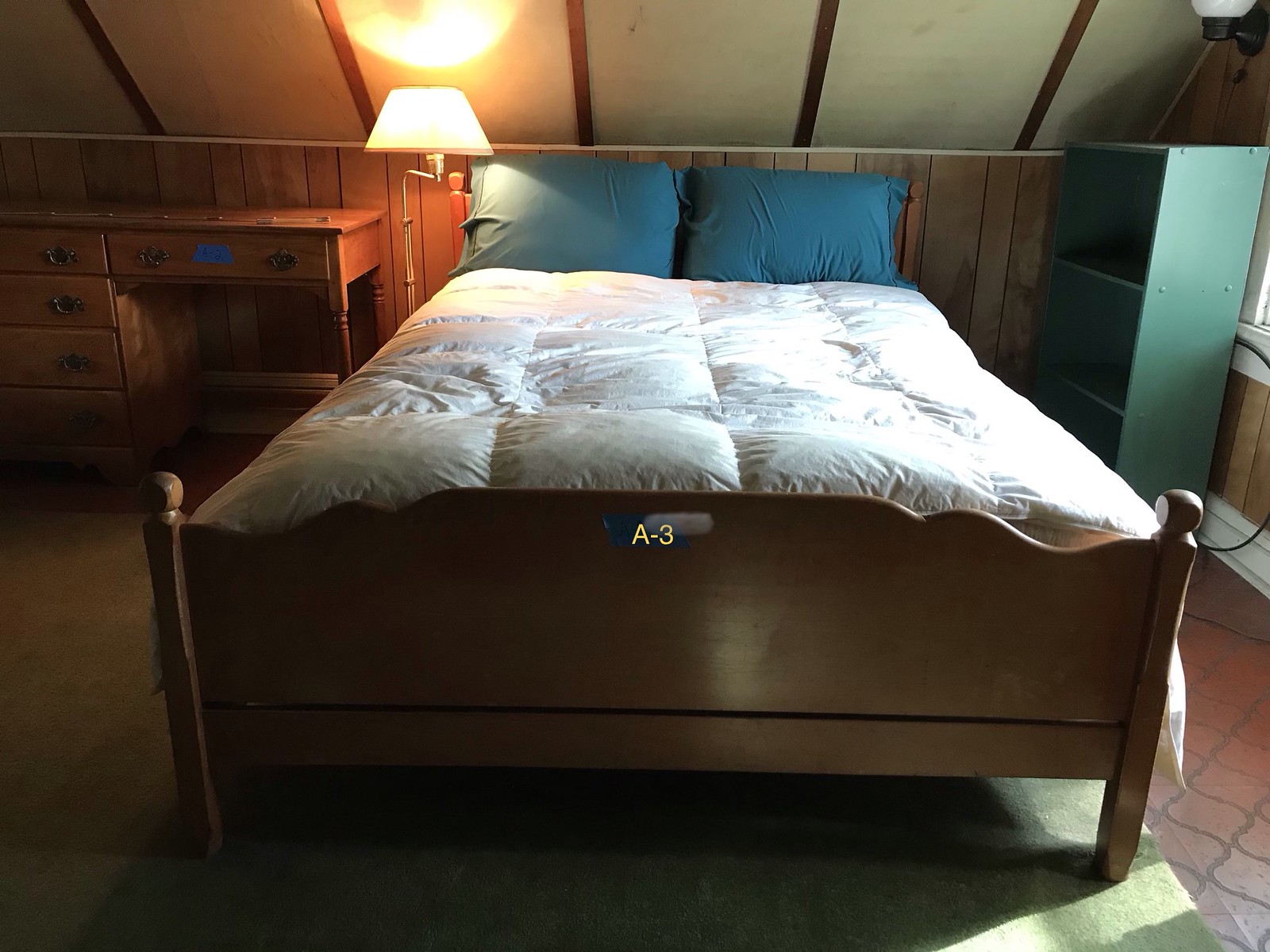The photograph captures a cozy attic bedroom, distinguished by the slanted roof visible at the top of the image, which hints at its location in the house. The focal point is a dark brown wooden bed frame, showcasing a prominent headboard and footboard, the latter embellished with the gold letters "A3" at its center. Draped over the bed is a pristine white quilt comforter, complemented by two dark blue rectangular pillows placed at the head. The right side of the image reveals a narrow rectangular set of green shelving, offering some storage space. Nearby, a floor lamp with a white shade casts a warm glow across the room, illuminating a small wooden desk and chair positioned to the left of the bed. The floors give off a rustic charm with their dark brown tile finish, partially covered by a green carpet that adds a touch of color and warmth to the space. Overall, the room emanates a quaint and homey atmosphere, bathed in gentle light filtering through an unseen window.